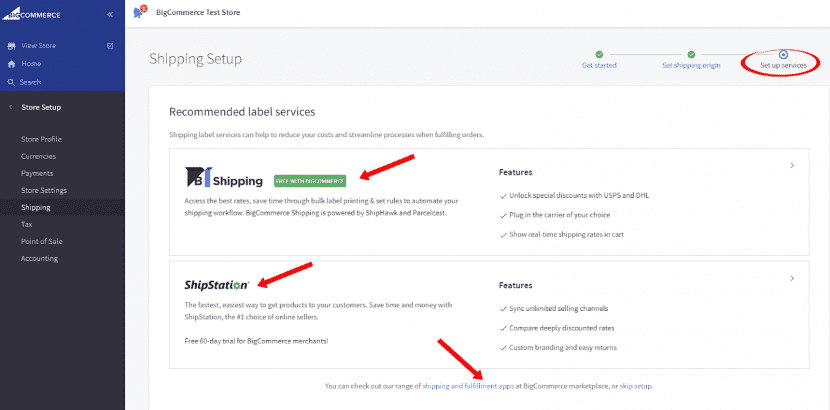This image appears to be a detailed screenshot of a user interface on a computer screen, likely from a commerce-related platform. The left side features a vertical column, with the top segment colored blue, containing the label "Commerce," and the lower three-fourths of the column colored black, displaying the text "Start Setup." To the right of this column, there is a predominantly white area.

In the upper left corner of the white section, the title "Big Commerce Test Store" is visible. Below this, a gray subsection titled "Shipping Setup" is present. On the far right side of the screen, the text "Setup Services" is highlighted and circled in red.

In the middle left of the white area, there is a section labeled "Recommended Label Services." The first entry under this heading is "Shipping," next to which lies a green button pointed to by a red arrow. The text on this button is not legible due to small font size.

Further down, there is a section titled "Ship Station," which is also indicated by a red arrow. At the very bottom of the image, a note says, "you can check out our range of Shipping and Fulfillment Apps," with the phrase "Fulfillment Apps" specifically pointed out.